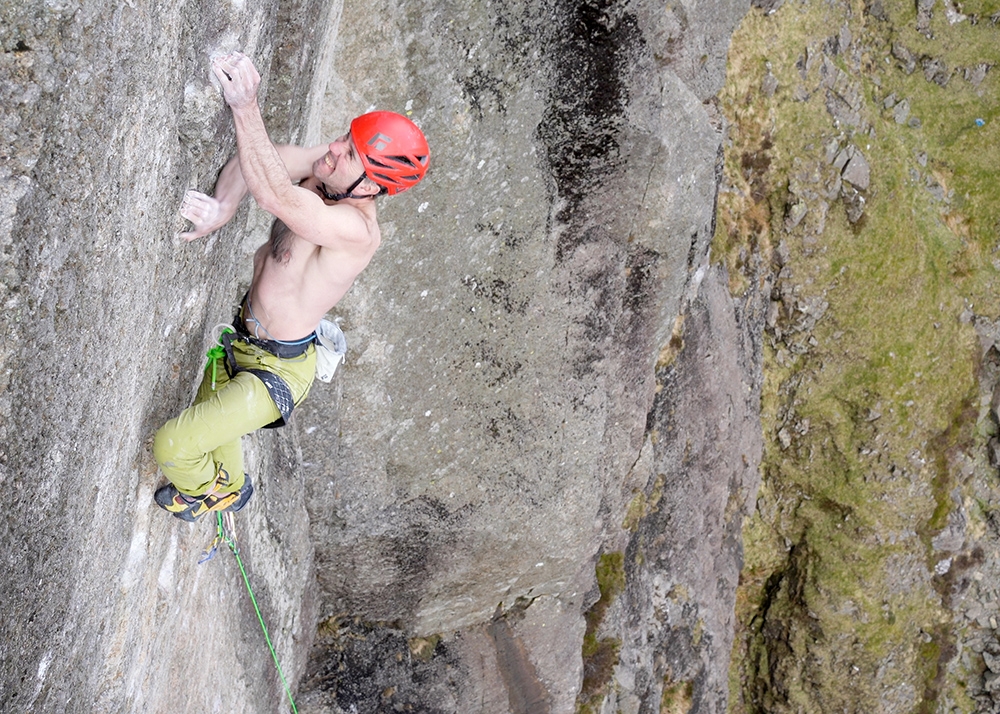The image showcases a shirtless, muscular rock climber on the left-hand side of a sheer, vertical gray granite cliff, dotted with black patches and small crannies. The climber, a young Caucasian man in his 20s or early 30s, is intensely focused, gripping the rock face with both hands; his left arm is raised higher than his right, which is bent. He sports an orange helmet with a black strap under his chin and is secured by a green rope attached to a carabiner on his belt. His lime-green pants and black-and-yellow climbing shoes stand out against the rugged backdrop. Below him, the rock face extends downward, meeting a mix of rocky debris and green moss at the base. The photograph is slightly angled from the side, suggesting the presence of another climber or observer, and captures the steepness and verticality of the climb, emphasizing the climber's bravery and determination.